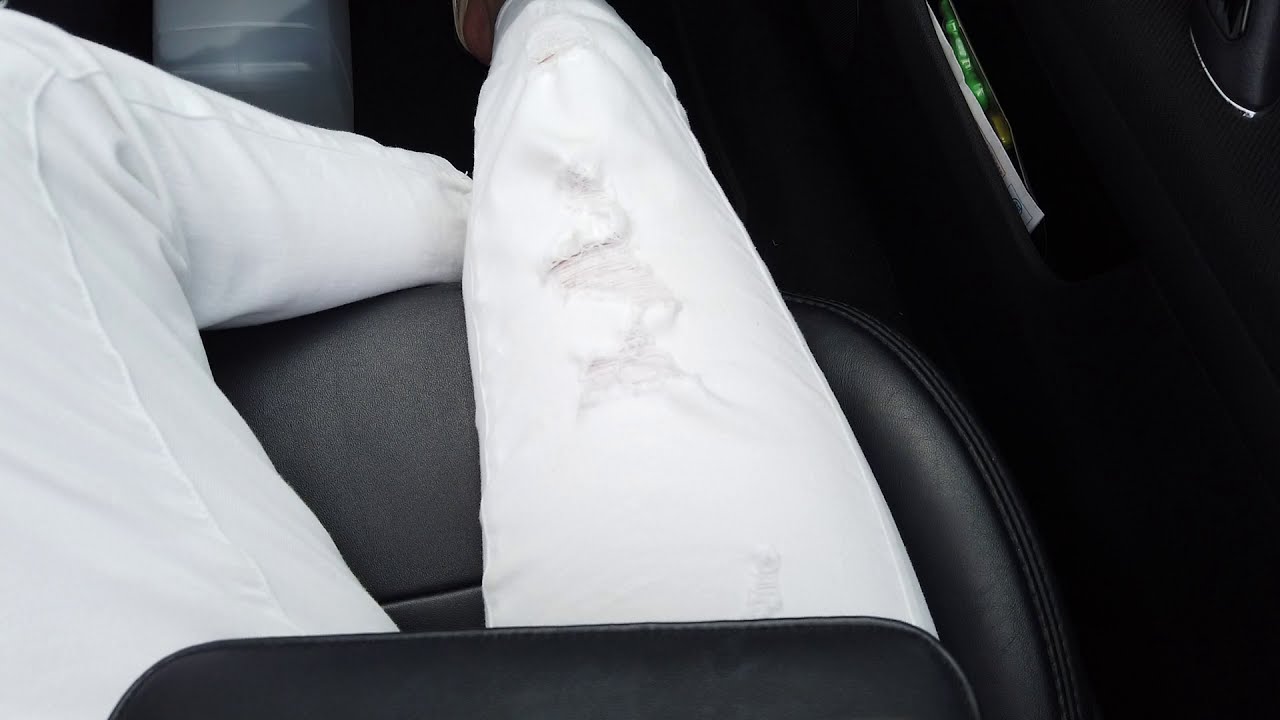Inside a vehicle, this image captures a person's legs adorned in white pants. They are seated on a black leather bucket seat. Their left leg is slightly opened to the left, forming a triangle with the right leg and the seat below. The main focus is the right leg, which has a noticeable gray zigzag smear, suggesting it brushed against something dirty. The seat they are on is visible within the triangular gap formed by their legs, and a portion of the black interior door can be seen to the right. The door compartment contains papers of white, green, and yellow hues. At the bottom of the image, the person's right heel peeks out from an open-toed shoe, and to the left, there's a plastic jug lying on its side filled with clear liquid, likely water. The overall lighting emphasizes the legs and the smudge on the pants, while the rest of the image remains relatively dark.